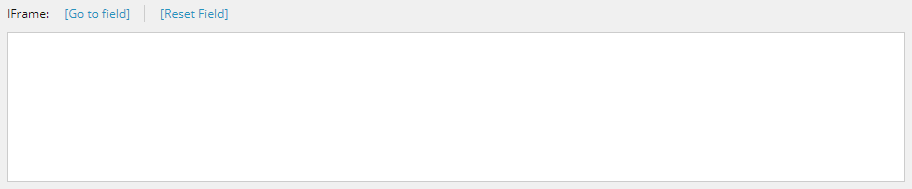The image features a rectangular layout with a light gray border surrounding the entire rectangle. A slightly thicker banner or border appears at the top. In the top left corner of this banner, the text "IFramed:" is displayed in a single word with a capital "I" and "F." 

To the right of this text, there are blue brackets enclosing the phrase "Go To Field," with each word capitalized. A fine gray line divides the image horizontally, and to the right of this line, more blue brackets enclose the text "Reset Field," where "Reset" and "Field" are both capitalized.

The background of the rectangle is plain white with no additional images, graphics, or text beyond what has been described.